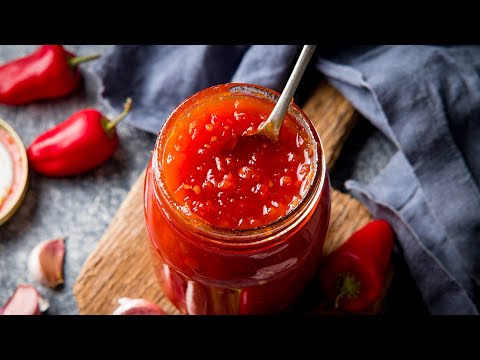The image showcases a glass jar of finely chopped salsa, positioned as the centerpiece atop a wooden handheld cutting board. The jar is open, revealing the salsa's mixed contents, with a spoon protruding from the top. To the left of the jar, two bright red chili peppers with green stems are placed beside the board, along with several cloves of garlic—one on the board and two just to the left. A single red chili pepper lies on the cutting board to the right of the jar. The setup rests on a bluish cloth that covers the table surface, adding a contrasting background to the scene. Additionally, a white plate with a floral pattern around its rim is partially visible on the left side of the image. The photo has black borders on the top and bottom, suggesting it has been cropped, and the setting appears to be on a stone or granite countertop.